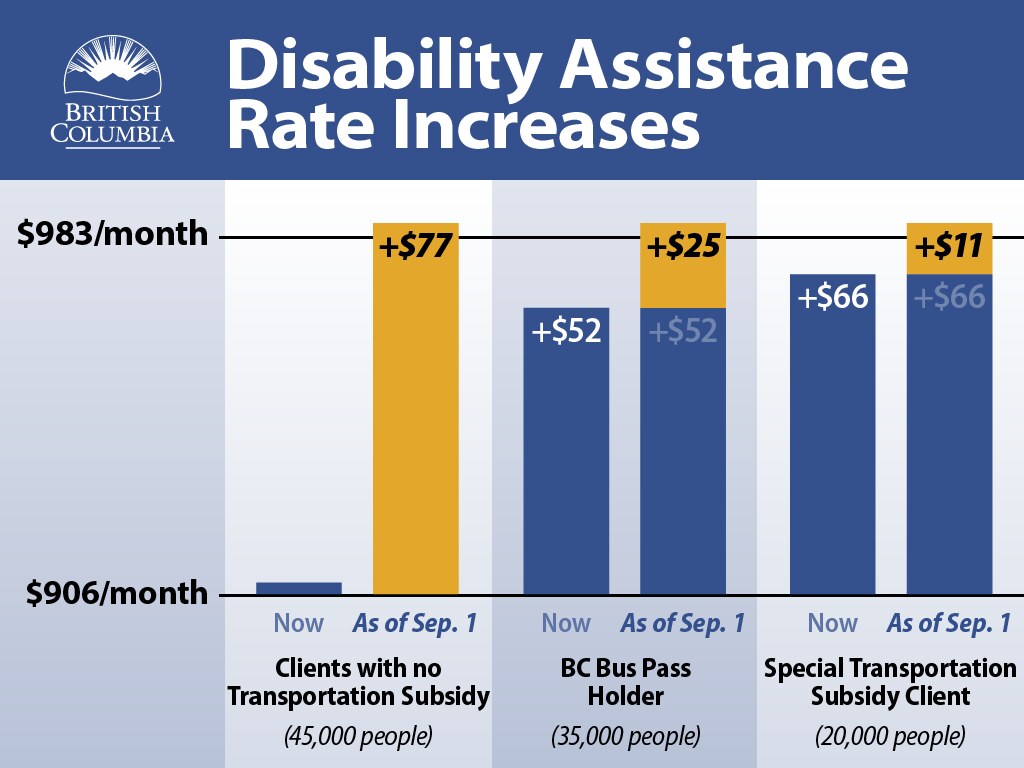The image is a detailed bar chart illustrating Disability Assistance Rate Increases in British Columbia. At the top, a horizontal blue strip reads "Disability Assistance Rate Increases" in white text, alongside a logo of a rising sun over mountains with "British Columbia" in white letters underneath. Three sections divide the bar chart, each representing different categories of clients and their monthly financial assistance.

On the left, the first section is titled "Clients with No Transportation Subsidy" and notes serving 45,000 people. It features a small blue bar marked "+$0" for the current rate, and a significantly taller yellow bar labeled "+$77" marked "As of September 1," which indicates an increase from $906 to $983 per month.

The middle section, "BC Bus Pass Holder," catering to 35,000 people, includes two blue bars, both labeled "+$52," with the current and added amounts overlayed, alongside a shorter yellow bar stacked on top adding an additional "+$25" for a total increase from $906 to $983 by September 1.

The right section, "Special Transportation Subsidy Client," representing 20,000 people, shows a blue bar labeled "+$66" for now, and another blue bar indicating "+$66" plus a yellow bar on top marked "+$11" for a combined increase reaching $983 as of September 1.

Horizontal black lines demarcate the current and new monthly assistance rates of $906 and $983, respectively. This comprehensive graphical representation highlights the specific rate increases and the population segments benefiting from the enhanced disability assistance provided by British Columbia.